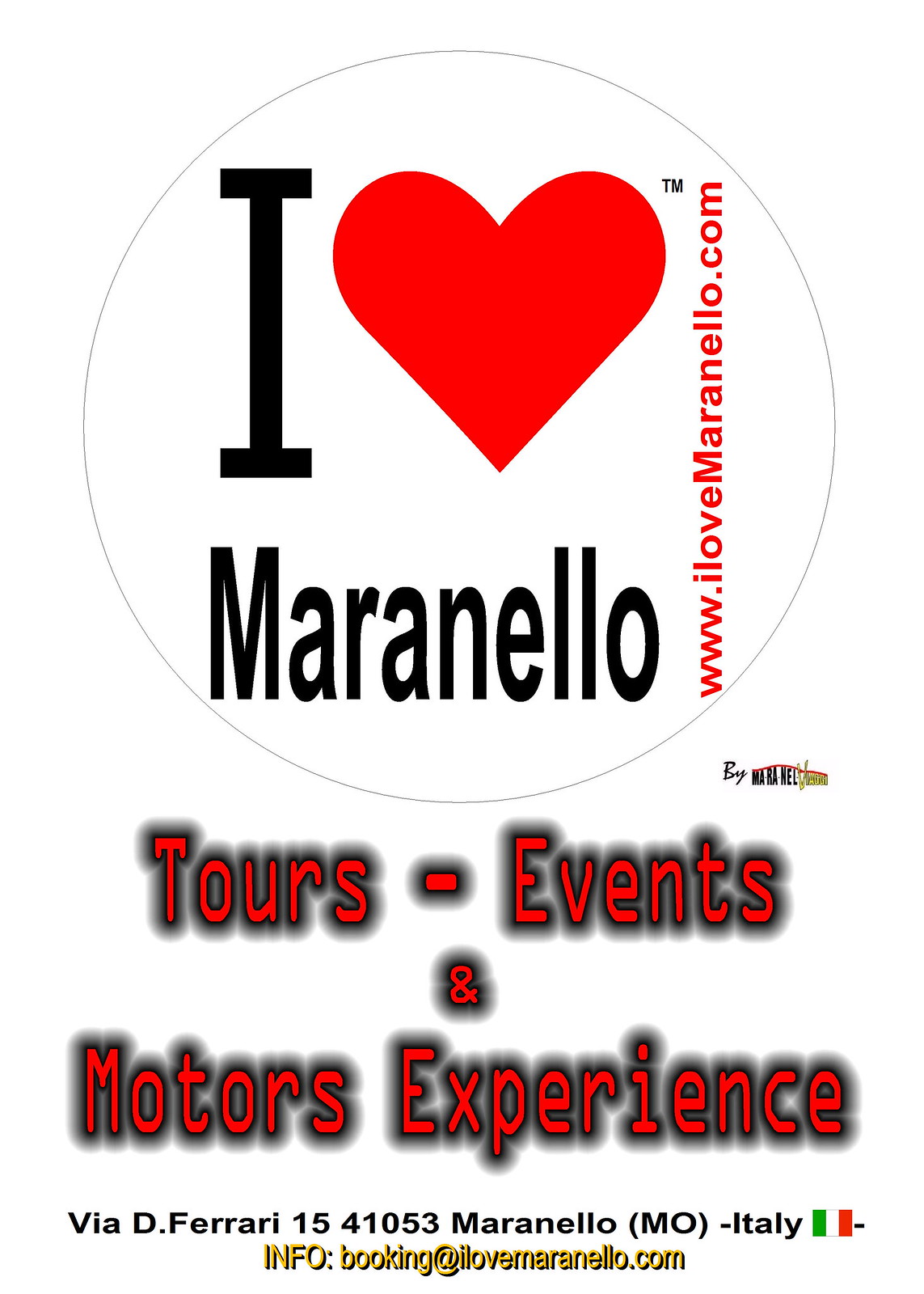The image is an advertisement with a white background, featuring a prominent white circle with a thin black border. Inside the circle, it says "I ♥ Maranello," where the heart is a red symbol. Displayed to the right in red text is the web address "www.ilovemaranello.com." Below this, also in red text, it reads "Tours, Events, and Motors Experience." Further down in black text, the address "via D.Ferrari 15, 41053 Maranello, Italy" is visible, with "MO" in brackets and accompanied by a small Italian flag showing green, white, and red stripes. In yellow text, it reads "Info, Booking at ilovemaranello.com." Additionally, there is a logo that is somewhat difficult to see, which helps identify this as a promotional flyer for a service offering tours, events, and motors experiences in Maranello, Italy.